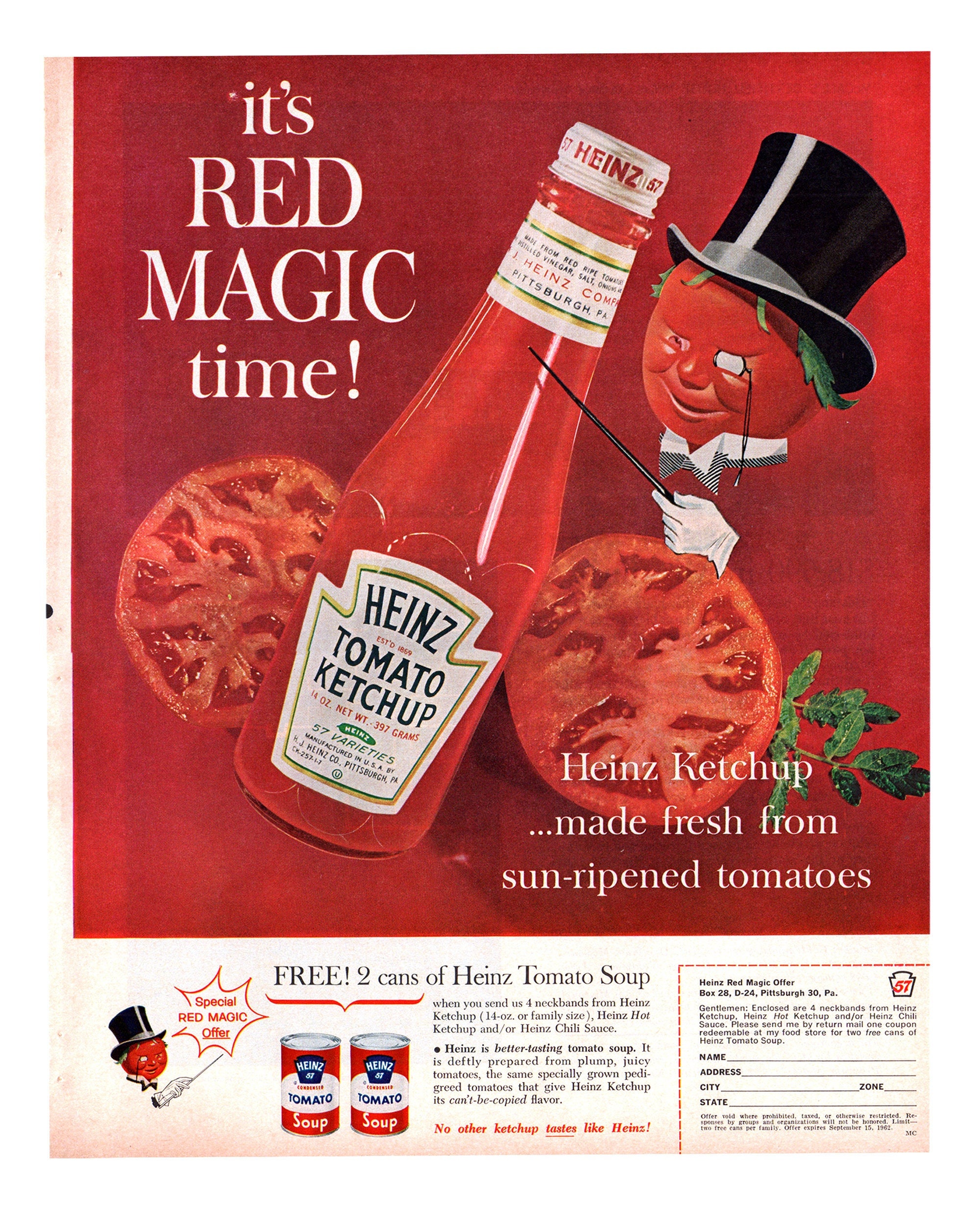This magazine advertisement for Heinz Tomato Ketchup features a bold, red background with a light beige trim along the left and bottom edges. Dominating the center is a sealed bottle of Heinz Ketchup, flanked by two halves of a sliced tomato. A quirky tomato character, dressed with a black top hat, green leaves sprouting underneath, and a tuxedo-style bow tie, stands prominently. This character, with white gloves on his hand, points to the ketchup bottle with a pointer stick. At the top of the poster, bold text reads, "It's red magic time," while a smaller subtitle below the bottle declares, "Heinz Ketchup made fresh from sun-ripened tomatoes." At the bottom of the advertisement, a special offer is highlighted: "Free two cans of Heinz Tomato Soup," accompanied by instructions for obtaining a coupon. The poster also includes spaces for users to fill in their name, address, city, and state to claim the offer.